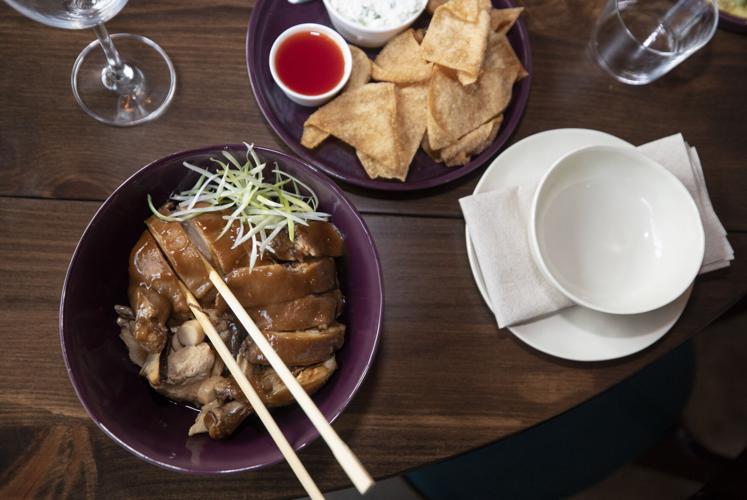This is an image of a dark wooden dining table with a rich grain pattern, set for what appears to be a Japanese or Chinese meal. In the bottom left corner, there is a burgundy bowl containing pieces of meat smothered in dark brown gravy, with wooden chopsticks sticking out. The dish is garnished with what seems to be white and green sprouts. Adjacent to it, slightly towards the center, a small wine glass and a transparent water glass frame the setup. 

Central to the table, there is a purple-burgundy plate holding what looks like fried wontons or chips, accompanied by two dipping sauces: a red sauce in a small white container and a white sauce in a slightly larger white container. Positioned to the center right, there is a white plate topped with a neatly folded white napkin, and a white bowl rests atop the napkin. The tableware is predominantly purple and white, providing a striking contrast against the dark wood surface, creating an inviting and elegant dining experience.